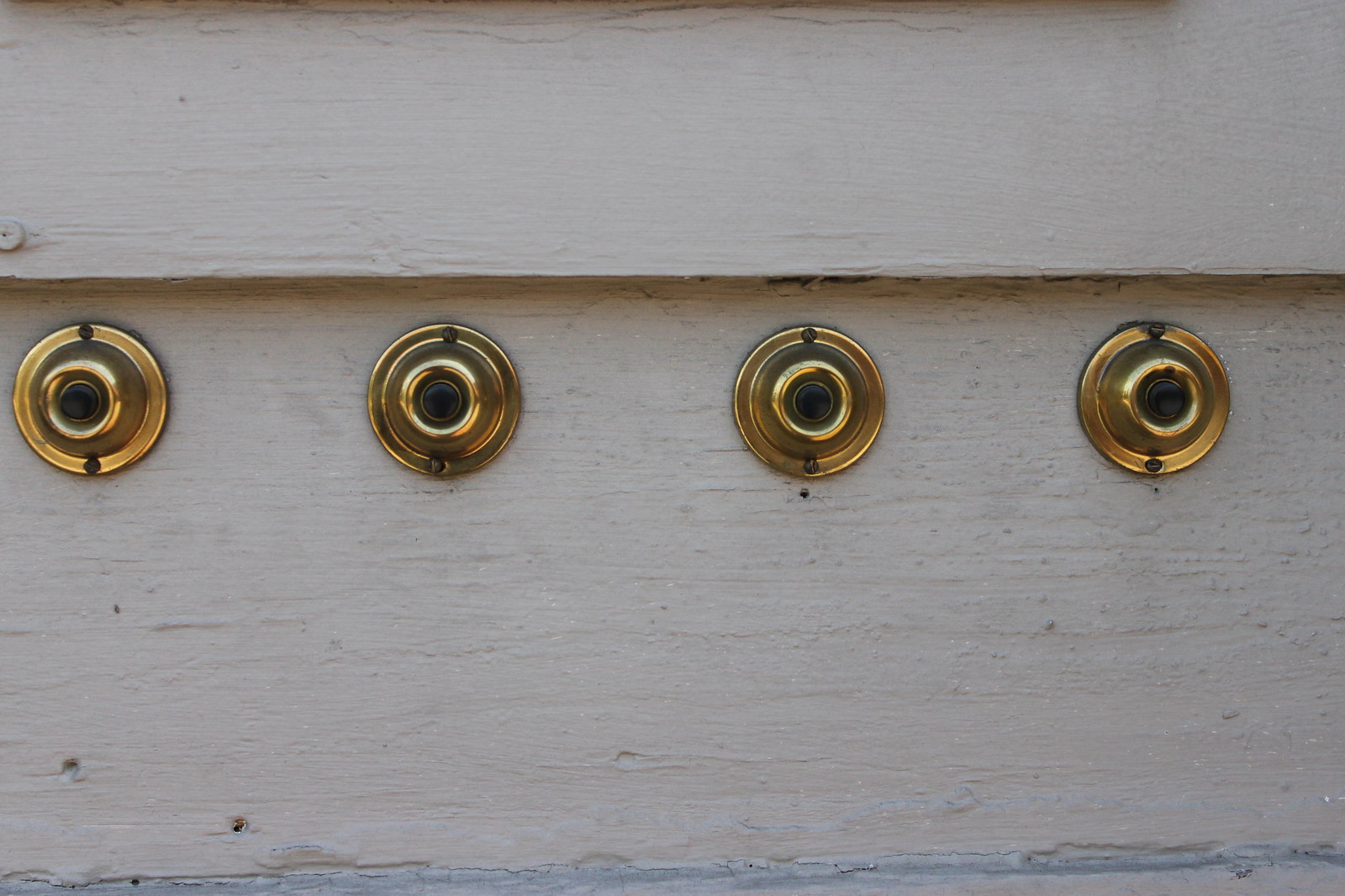This photograph depicts four shiny brass doorbells evenly mounted on a horizontal piece of timber, painted in a creamy beige hue that resembles house siding or clapboard. Each doorbell features a circular brass housing with a flat, disc-like appearance, accented by a slightly raised outer ring. In the center of each disc is a black button, surrounded by a further raised ring. The brass plates are secured with screws positioned at the 12 o'clock and 6 o'clock points, contributing to their polished and possibly newer look. The image suggests an outdoor setting, but it leaves some ambiguity regarding whether the doorbells are functional or simply for display. The overall scene is a simple yet detailed showcase of neatly arranged, well-crafted doorbells against a subtly colored wooden background.